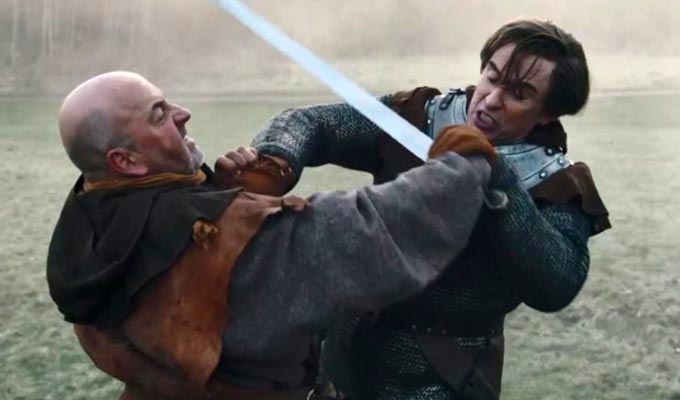In the image, we witness a vivid scene reminiscent of a medieval or Renaissance movie or TV show, where two men, clad in period attire, are locked in an intense struggle over a long sword. The duel takes place outdoors on a grassy terrain, with a backdrop shrouded in thick fog, giving a sense of impending storm or gloom. On the left stands an older, bald, Caucasian man dressed in heavy, friar-like fabric. His face bears a grimace as he contends with his opponent. Opposite him, on the right, is a younger Caucasian man with long dark brown hair, wearing a suit of armor, including chain mail and orange-brown gloves. He, too, is grappling fiercely, trying to gain control of the sword, his expression equally tense and frustrated. The absence of text ensures that the viewer's attention remains solely focused on the dramatic physical and emotional conflict between the two characters.